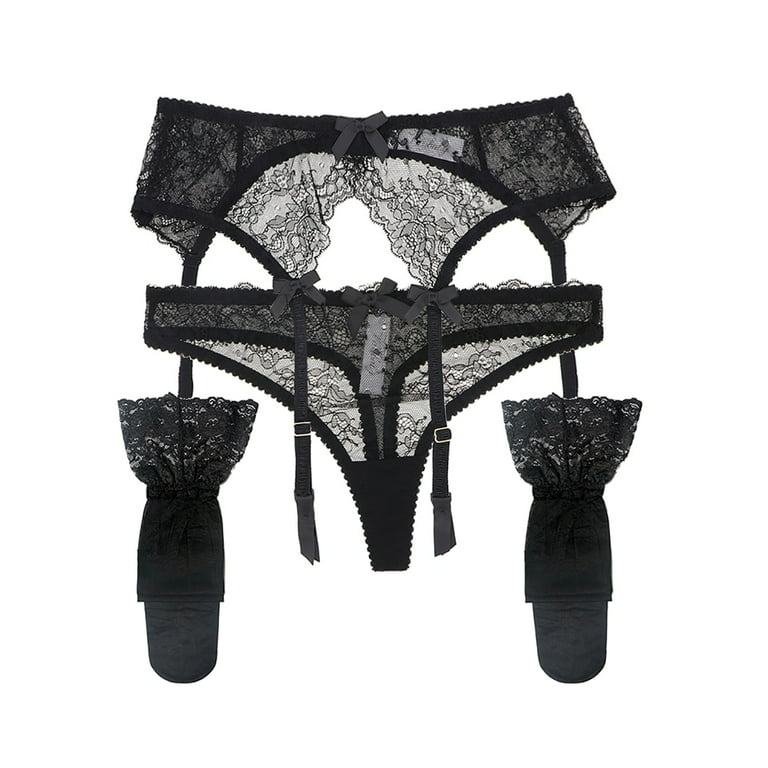This photograph features an intricately detailed set of black lacy lingerie elegantly arranged against a white background. The set includes a delicate black lace g-string thong, characterized by scalloped edges and a small black ribbon bow adorning the front. Complementing the thong is a matching garter belt, which also features scalloped lace edges and a central bow. The garter belt comes with two stockings, each meticulously folded to prevent damage, with broad lace tops that mirror the delicate, floral lace pattern of the other pieces. The overall design of the set exudes femininity and sophistication, enhanced by subtle silver detailing on the buckles and the visible, though unreadable, labels inside the garments. The refined craftsmanship of the lace and the harmonious arrangement of elements make this a striking and elegant ensemble.